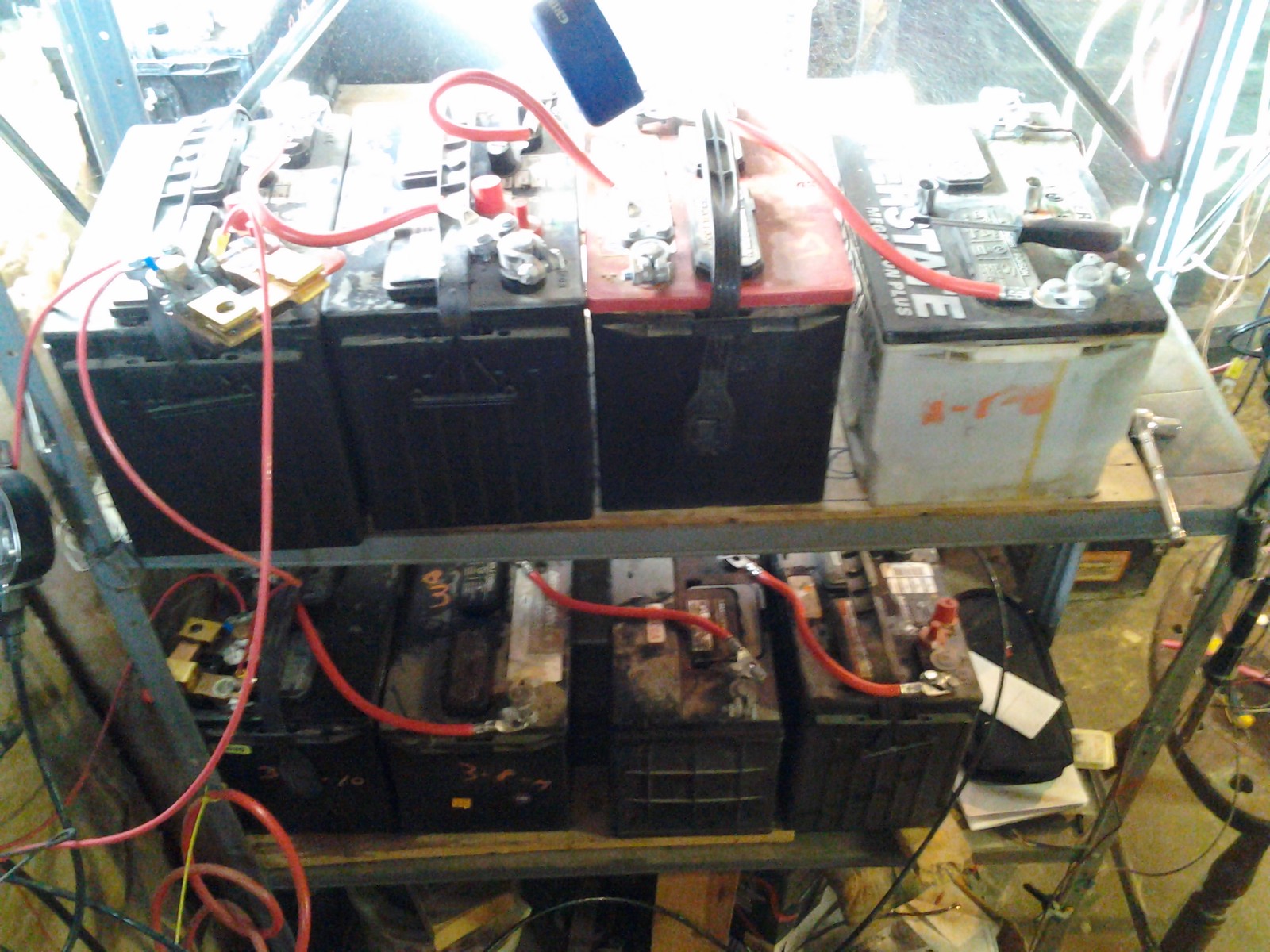This rectangular landscape photograph captures a shelving unit in what appears to be the back of a garage or car repair shop. The shelving, composed of silver metal bars and wooden shelves, stands three tiers high, though the bottom shelf may actually be the ground as it is barely visible. 

Positioned prominently in the image are several old and rusty vehicle batteries, indicating they have seen considerable use. The top shelf holds four batteries. The one on the far right is marked "Interstate" with a white body and a black top, while the second from the left features a red top; the other two have black tops. Connected by red cables, these batteries appear to be arranged for testing or recharging, with the cables extending towards the left side of the image. 

In the middle tier, the four visible batteries also show signs of wear, sharing the characteristic red cables connected to their terminals. On the right edge of the top shelf, next to the "Interstate" battery, there is a socket wrench, hinting at ongoing work in the space. 

In the upper background, there is an illuminated glass doorway, suggesting daylight shining through and adding a sense of depth to the workspace.